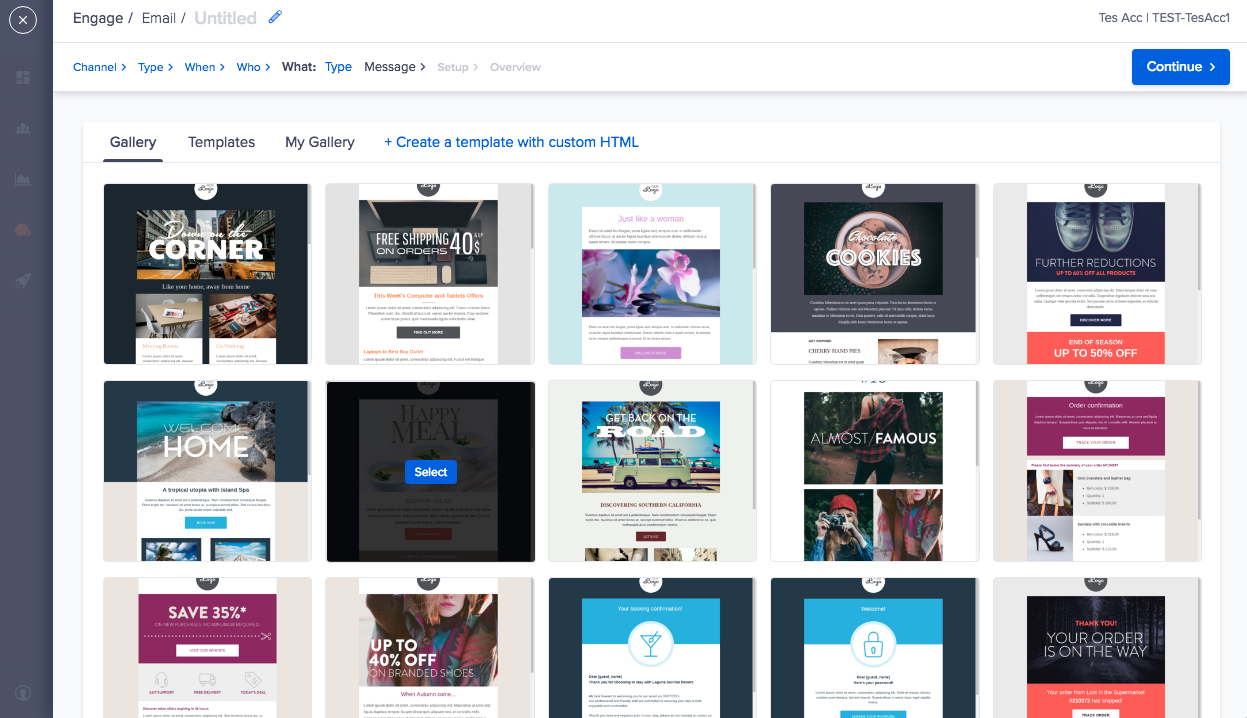In the image, to the left, there is a gray box followed by a faded image of a white circle with an "X". Next to this on a white background with gray lettering, it reads "engage / email / untitled". Adjacent to this, there's a blue pencil icon.

To the right, there is text that reads "test ACC" followed by a gray line and "test account". Below that, in a small blue font, it says "channel, arrow type, arrow when, arrow who". In black font, it says "what" and "message". In blue font, it says "type". Further right, very faded, it reads "set up" and "overview". Continuing to the right, there's a "continue" button in a blue box with white lettering and a white arrow pointing to the right.

Below this, in black font, it reads "gallery, templates, my gallery". In blue, it says "plus create a template with custom HTML".

On the left within a black outlined box and white lettering, it says "corner" with very tiny photographs. The next section with a gray background reads "free shipping" and "40s" in white. The next image has blue, almost square background, a white background with purple and gray lettering, a gray and purple image in the middle, and additional gray lettering inside the purple box.

Moving on, there's another gray box with black inside and white lettering that says "cookies" with an image of a brown cookie in a circle and white font underneath. Another image has a black background showcasing silver-gray shoes, white lettering, and red text below. Following this, there is a white background with gray lettering, a black box, an orange background, and white lettering.

The next line down has the word "home". It shows an unclear image that says "welcome home" in white font, with a gray background and blue on top, white background underneath with black lettering, and a blue box. Another image presents a faded gray background with a blue box in the middle with white text saying "select".

Further on, there is an off-white caravan image with the word "road" above it set against a blue sky with gray edges and black lettering underneath. Another image reads "almost famous" in white lettering with a distant photo background. Following this, there's an image with a pink background, a white box with white lettering, a light gray box below it, another white box that apparently has a pair of shoes, and a gray background.